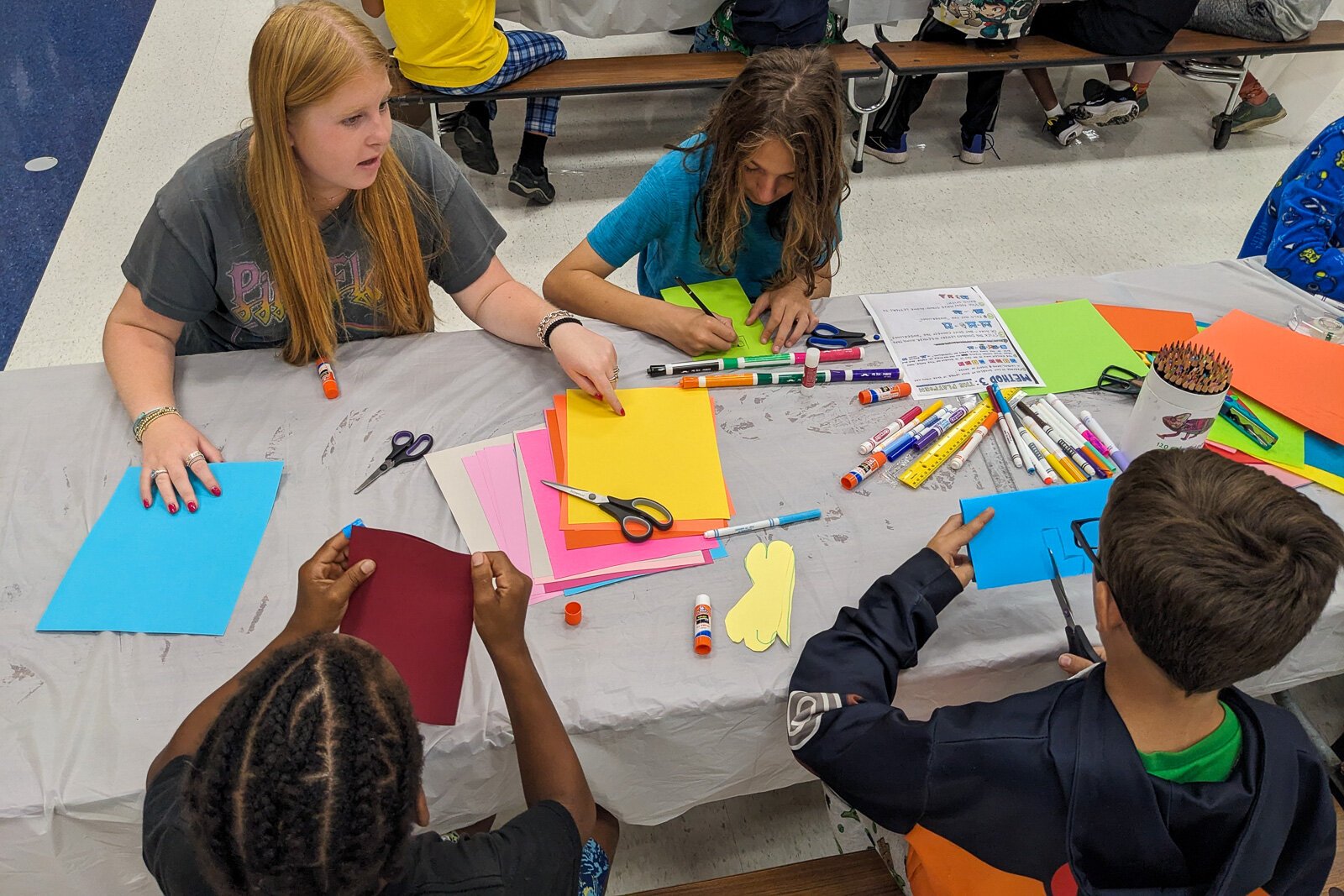In this image, a group of students and a probable teacher are gathered around a lunch table in what appears to be a classroom or cafeteria setting. The table is covered with cloths and scattered with various colorful pieces of construction paper as the children engage in an arts and crafts activity. 

On the left side of the image, an older woman, who might be the teacher, is involved in the project. She has long hair, red-painted fingernails, and is wearing a gray shirt with indistinct purple lettering. Her focus is on a piece of blue construction paper under one hand, while her other hand is touching a yellow paper. 

Next to her, a girl in a blue shirt is writing on a lime green paper with what seems to be a black pen. 

On the bottom right, a young boy with glasses is concentrated on cutting a piece of blue construction paper. He is wearing a dark blue hoodie.

Nearby, to the left, another child, whose gender is not clear, is folding a dark red maroon piece of paper and has a blue band-aid on the tip of one of their fingers.

Overall, the image captures the engrossed expressions of the children as they meticulously work on their creative projects, guided and assisted by the older woman.